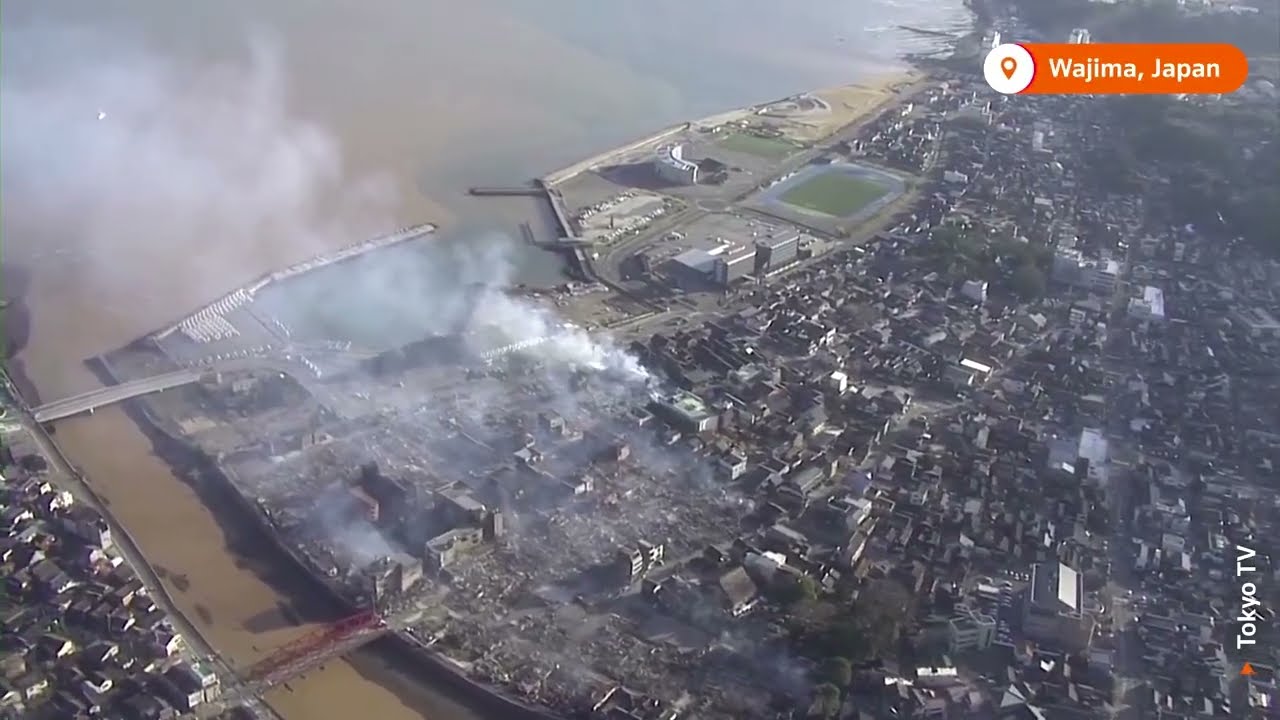This aerial photograph, attributed to Tokyo TV as indicated by the watermark on the lower right, captures a detailed view of Wajima, Japan. Dominating the upper right of the image is an orange rounded rectangle with white sections, featuring a location symbol and the name "Wajima, Japan." The shot is taken from an altitude of several hundred feet, providing a broad view of this coastal town. A murky brown waterway with two vehicular bridges connects the left portion of the city to the larger right portion, suggesting a network of interconnected areas.

In the center of the photo, a significant amount of white smoke is visible emanating from a building, possibly indicating a fire or a factory releasing emissions, though no flames are explicitly seen. This thick plume of smoke extends across a substantial part of the left half of the image. Adjacent to the area of smoke, there is a large athletic field, adding to the urban details. The upper left portion of the image reveals a body of water, potentially a bay or ocean, highlighting Wajima's coastal nature. The cityscape below includes numerous houses and buildings stretching back from the waterfront, painting a comprehensive picture of the town and its immediate surroundings.